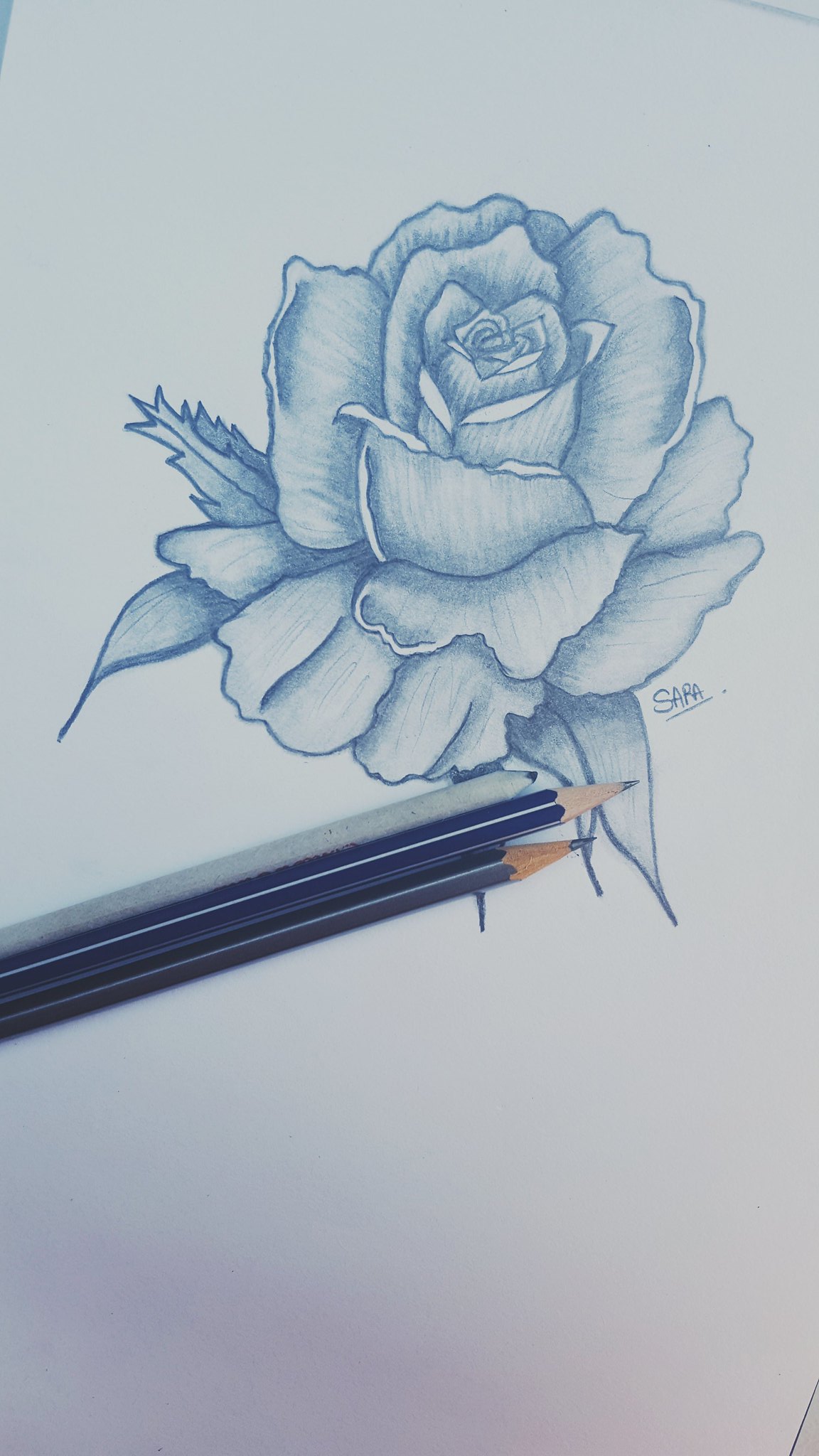This beautifully detailed image, seemingly crafted with colored pencils, prominently showcases three distinct pencils lying across the artwork. The first pencil, with a predominantly black body and a darker wooden end, reveals its deep blue shading material at the pointed tip. The second pencil appears almost like a dark royal blue or purplish hue, influenced by the lighting source. The third pencil stands out with a body that resembles a composite material, featuring a blend of white, blue specks. 

The drawing itself portrays a rose intricately shaded entirely in various tones of blue, including the green leaves below the rose that are also shaded with blue hues. Adding a personal touch, the name "SARAH" is inscribed in all caps in the lower right corner, underlined with a dot at the end. The image sits on a white piece of paper, which subtly transitions into light pink, light purple, and slightly bluish hues from the lighting, creating a gentle gradient effect towards the bottom of the paper.